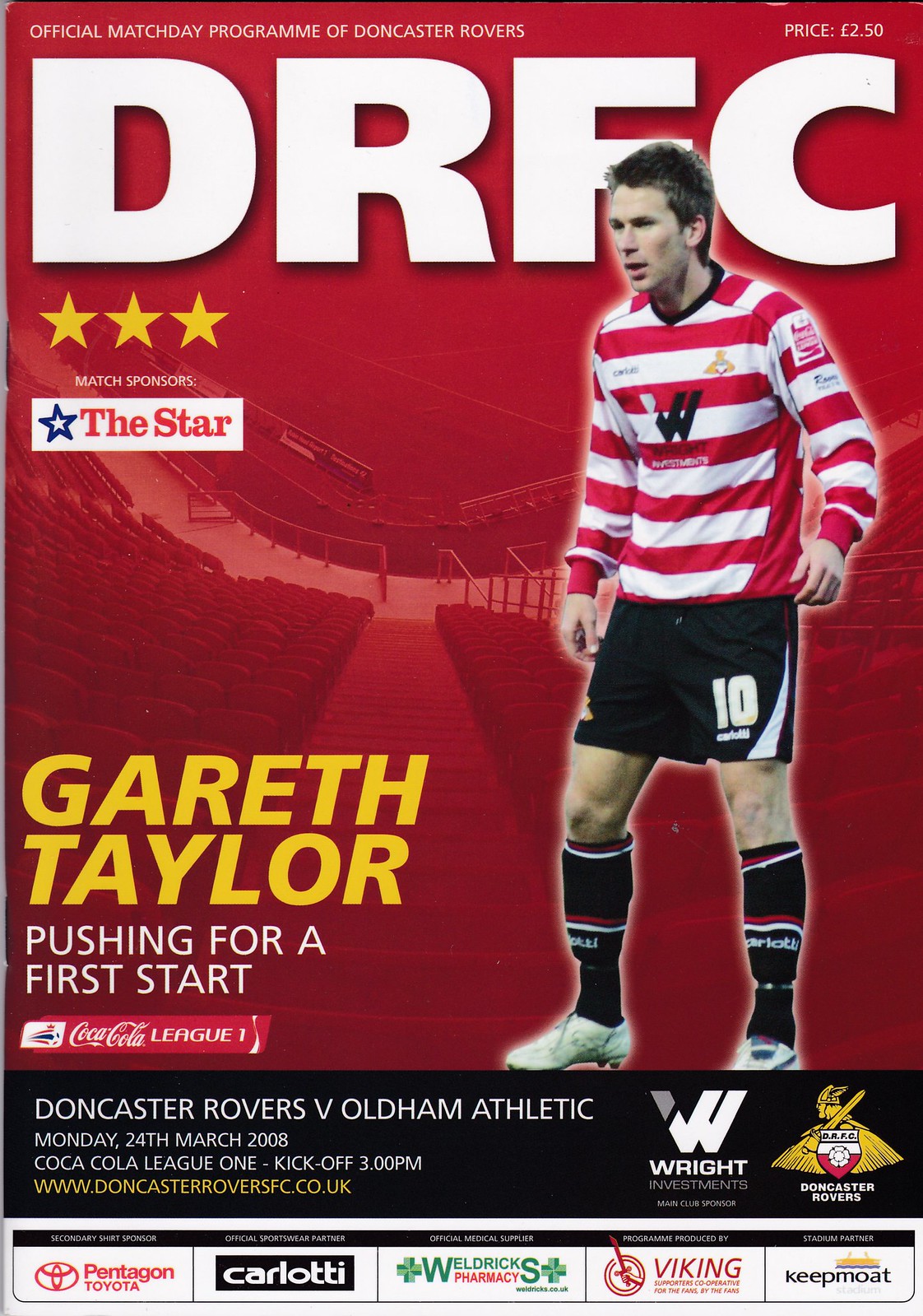The front cover of the official match day program for the Doncaster Rovers Football Club (DRFC) prominently displays a textured red background, which features a blurred image of a football stadium. At the top edge, in smaller text, it reads "Official Match Day Program of Doncaster Rovers," adjacent to the program's price of £2.50 located in the upper right corner.

Centrally placed in bold, white letters is the magazine's title, "DRFC", just below which are three gold stars. The cover also highlights the text "Search Sponsors" in white, and features an image of a soccer player, Gareth Taylor, standing in a red and white striped jersey with black shorts adorned with the number 10 in white, tall black socks, and white cleats. The player is positioned more towards the right side of the cover, facing left with his hands to his sides.

In the lower-left corner, Gareth Taylor's name appears in large yellow lettering, accompanied by the phrase "Pushing for a start" in white. Below this, the text "Doncaster Rovers versus Oldham Athletic, Monday, 24th March 2008, Coca-Cola League One, kickoff 3 PM" is prominently displayed on a black strip running across the bottom. The Doncaster Rovers' website, www.doncasterroversfc.co.uk, is also included here.

The cover is dotted with several sponsor logos and names, including Coca-Cola in a red banner, Pentagon Toyota, Carlotti, Weldrick's Pharmacy, Viking with a logo featuring a circle with a hand holding a sword, and Keep Moat, which features a logo of a moat. Additionally, the Doncaster Rovers' crest, which consists of a shield set against a gold triangle, is displayed on the right side of the black banner at the bottom of the page.